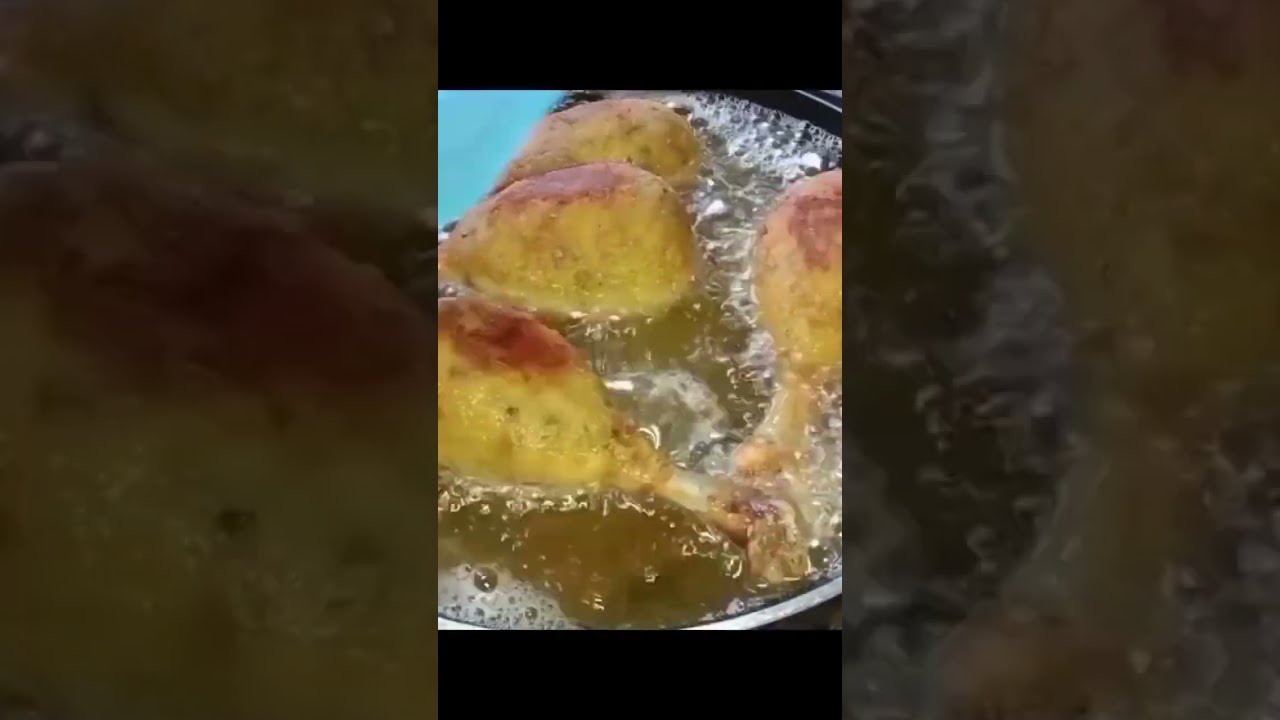The image is a close-up shot of chicken drumsticks, likely taken from a camera phone, showing four drumsticks floating and boiling in hot oil. The oil is a yellowish, bubbling liquid that occupies the center of a circular pot, which we are looking down into. The drumsticks have a tannish, goldish color with darker brown spots, indicating they have been rotated and cooked. Some drumsticks have bones sticking out, especially noticeable on the bottom right. The image has been cropped vertically, with black borders at the top and bottom, and it has a shadow effect on the left and right, making it appear larger. There's a hint of something blue, possibly a utensil, in the upper left corner. This detailed close-up, which may be a screenshot from a cooking video, highlights the textures and colors of the frying process, with the skin of the drumsticks being lightly browned and greasy, suggesting a potentially indulgent meal.